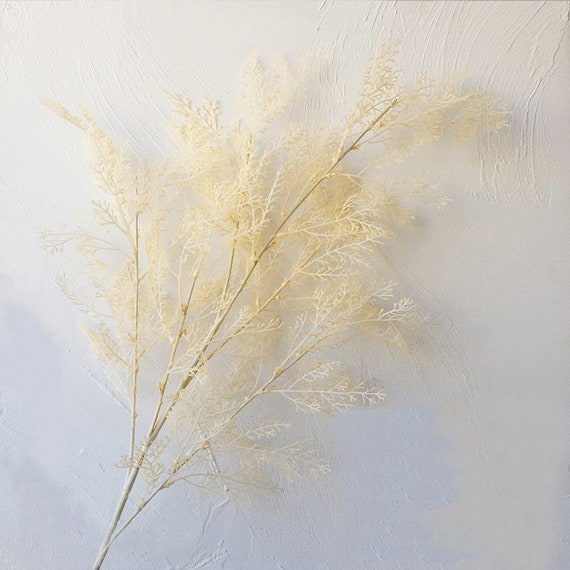This image showcases a piece of minimalist artwork featuring a branch with delicate, feather-like leaves. The branch, a very light tan or almost golden color, stretches diagonally from the bottom left to the top right, resembling the spread of a fan. The leaves, in shades of white, cream, and subtle hints of yellow, blend softly with the cloudy white background, which has a textured and somewhat blurred appearance. At the bottom of the artwork, the background takes on a light gray hue, giving more definition to the base of the branch. The textured background features swirling lines, adding an artistic touch to the piece. The interplay between the branch and its blurred, subtly colored surroundings creates a serene, almost snow-like visual effect, enhancing the overall ethereal quality of the image.